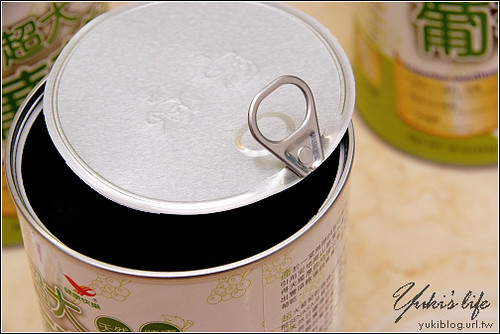The photograph features a prominent open can of food at the center, set against a pinkish marble surface. The can has a yellowish-white label with an image of grapes, and its silver lid is partially peeled back, revealing a solid black interior. Chinese characters are engraved on the can, and paragraphs of black text, likely nutritional information, are visible on the back. Behind the central can, there are two more cans with green and yellowish-white labels adorned with green Asian characters. In the bottom right corner, a cursive inscription reads "Yuki's Life, Yuki Blog, URL TW," adding a personal touch to the image.